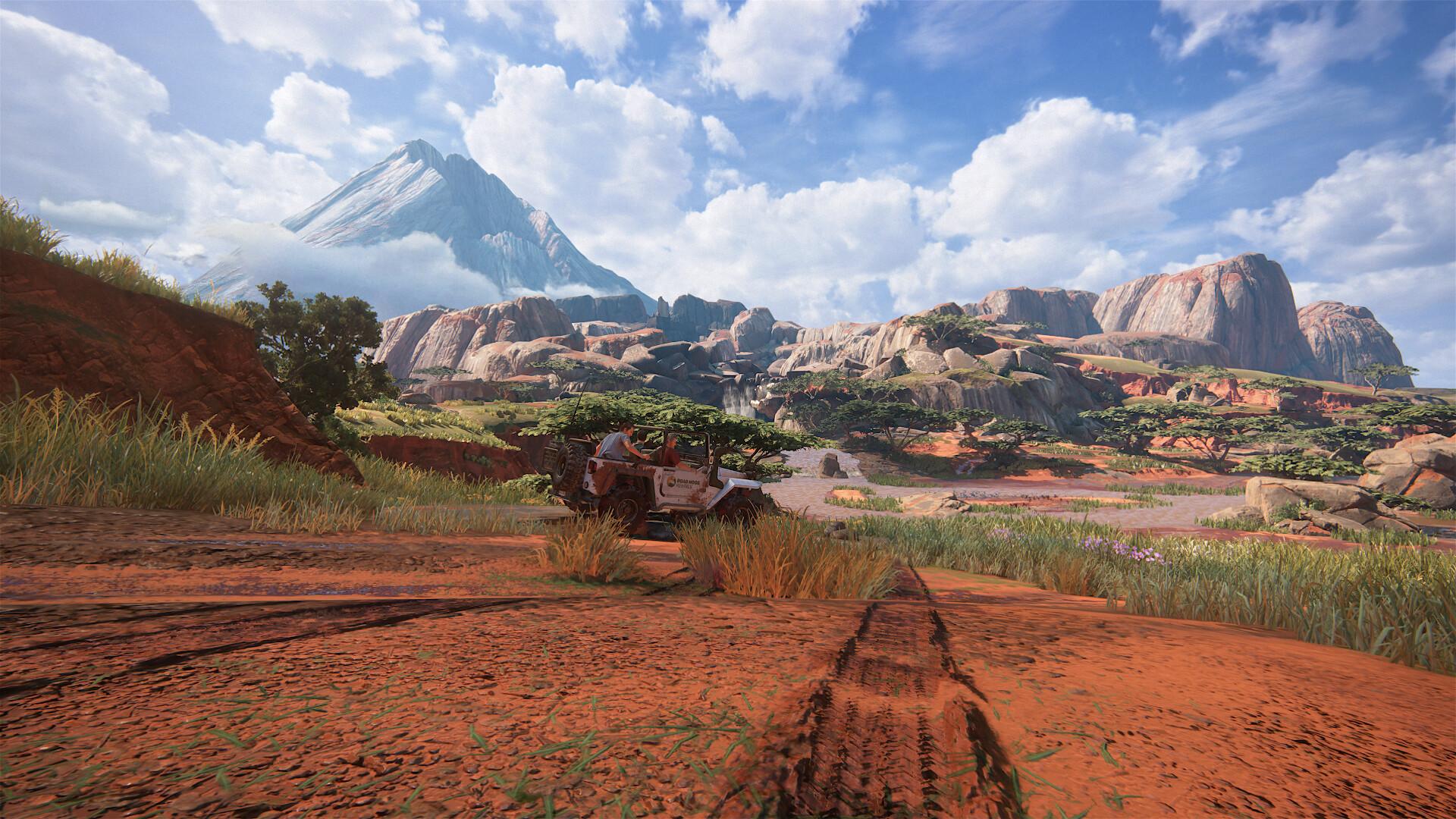In the image, a desolate desert landscape stretches out before the viewer, evoking a sense of isolation. The terrain, which appears to be computer-generated, features reddish clay-like dirt that dominates the scene. Prominent among the features is a large tire track that cuts through the earth, suggesting a recent passage of a heavy vehicle. Scattered patches of wild grass and weeds struggle to thrive in this harsh environment, adding a touch of green to the otherwise stark scenery.

In the distance, a majestic range of snow-capped mountains towers over the horizon. Smoke or mist can be seen rising from the area around the peaks, adding a layer of mystery to the landscape. The left side of the image showcases elevated reddish dirt formations, contrasting with the lower, brown hills on the right. Above, the sky is overcast with clouds, yet rays of sunlight manage to break through, illuminating parts of the rugged terrain.